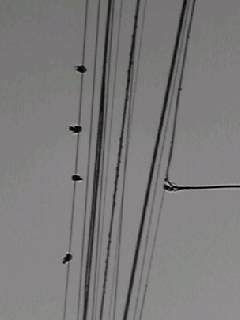A photograph captures a dark gray sky with several power lines crisscrossing from left to right. The viewer's perspective is from below, looking up at the web of cables. On the topmost and thinnest of these lines, five birds are perched, equally spaced, appearing as small black silhouettes against the murky backdrop. To the left, the thin line with the birds is paralleled by another thin line followed by a thick one. Moving right, this pattern continues with alternating thick and thin lines. A prominent pole can be seen entering from the right side of the image, supporting this intricate network of power lines. The scene offers a stark contrast between the stark modernity of the cables and the simplicity of the birds, all set against the somber gray tones of the sky.